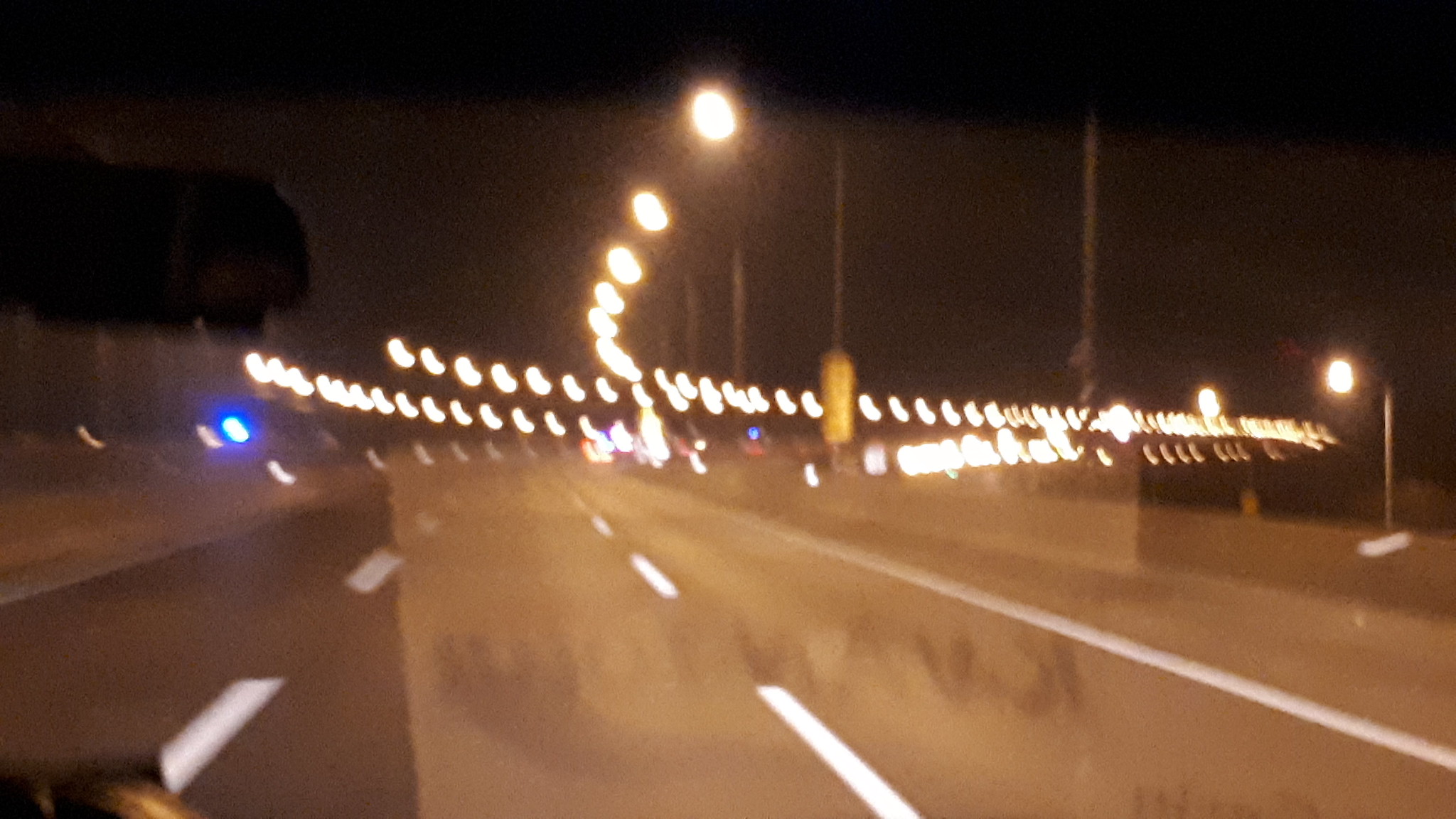A nighttime photograph captures a deserted freeway as seen from the windshield of a moving car. The image, though somewhat blurry due to the motion of the vehicle, shows the car traveling in the middle lane of a three-lane highway. Distant taillights barely break the darkness as they gleam faintly far ahead. Street lamps line both sides of the road, casting a soft glow on the empty asphalt. A small breakdown lane is visible on the right-hand side, complemented by a narrower emergency lane on the left. In the upper left corner of the photograph, the rear-view mirror is discernible, alongside an indistinct reflection in the windshield. A mysterious blue light is seen beyond the left-side divider, hinting at some sort of traffic signal or beacon in the distance. The overall scene is shrouded in the stillness and dim light of night.